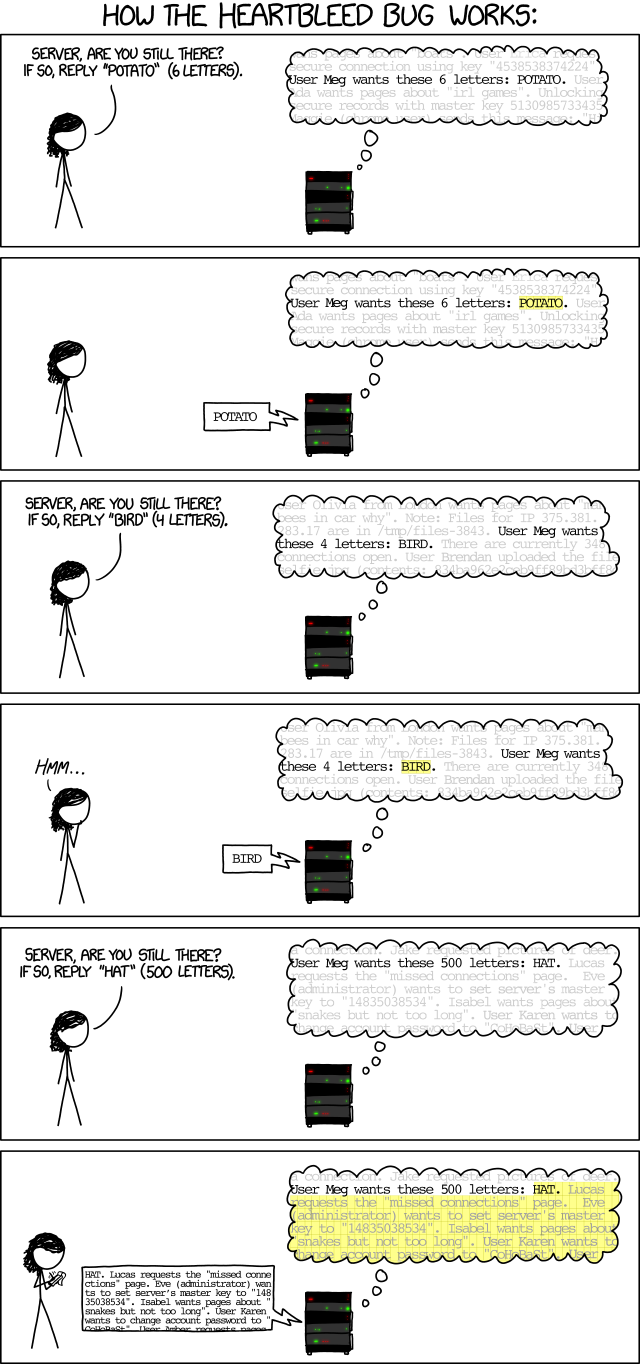Here is the revised and detailed caption:

---

In this technology comic titled "How the Heartbleed Bug Works," a female character interacts with a server stack. She starts by asking the server, "Server, are you still there? If so, reply 'potato', six letters." The server responds with "potato." She then asks, "Server, are you still there? If so, reply 'bird', four letters." The server replies with "bird." 

Curious, she tests the system further: "Server, are you still there? If so, reply 'hat', 500 letters." The server, due to a vulnerability, spills a significant amount of data beyond the 'hat' request. This data dump includes various system strings and crucial information such as the server's master key, "04822."

Through persistent probing, the woman takes advantage of the Heartbleed bug, an old but critical vulnerability that exposes sensitive server data. Observing the server's responses, she records potential passwords and other critical data that should have been protected, underscoring the severity of this security flaw.

---

This cleaner, more detailed caption captures the essence of the comic while highlighting the Heartbleed bug's exploitation process.